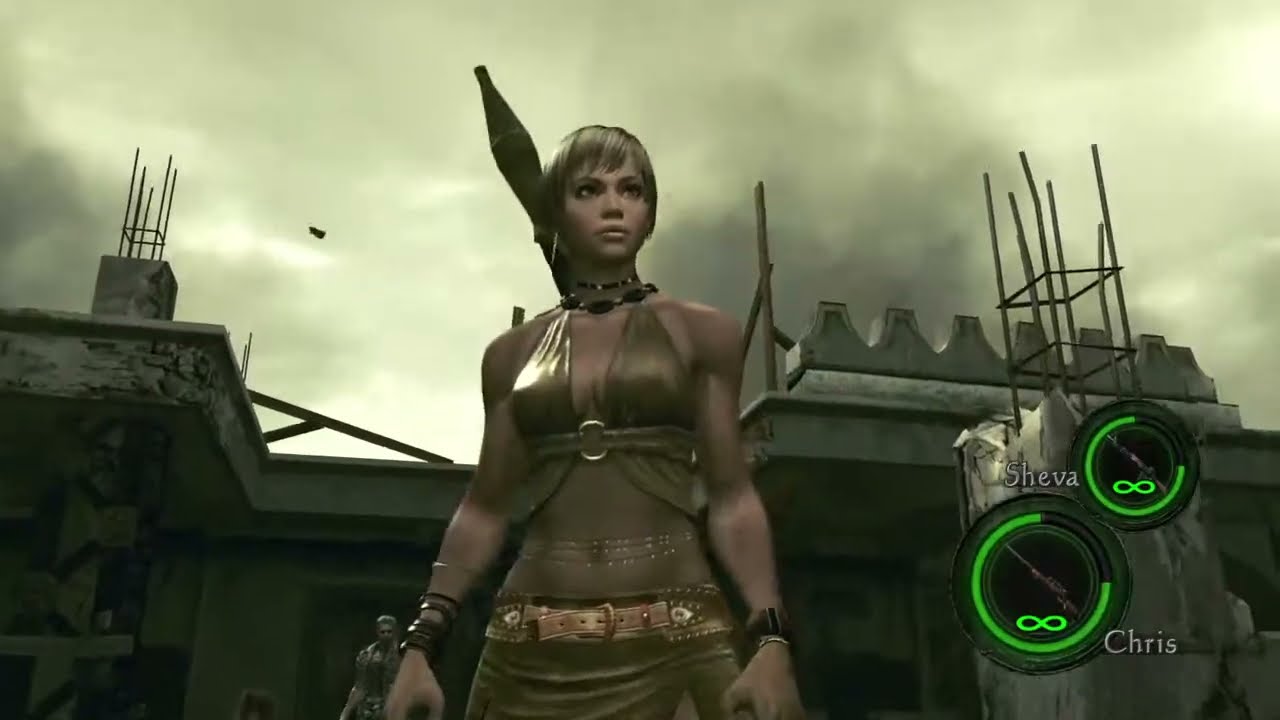This image is a screenshot from a video game, featuring a prominently centered, animated female character with tan skin and light brown to blonde hair. She is dressed in a striking gold ensemble: a halter top connected by a silver ring, exposing some cleavage, with gold chains wrapped around her midriff, and a matching gold skirt with a belt. She accessorizes her outfit with multiple black and gold bracelets on both wrists, and two black necklaces. The character has a stern expression and stands ready for a fight, with a grenade launcher or some sort of weapon over her right shoulder and what might be a weapon on her wrist. 

In the lower left corner of the screen, the names Shiva and Chris are displayed next to green rings, possibly indicating health or status in the game, with Chris being prominently highlighted. The background features a dark, gray sky suggestive of destruction, with what appears to be the remnants of a large structure resembling a demolished castle or fortress, characterized by parapet-like projections and metal reinforcements. There is also a small figure or silhouette in the distance, adding to the scene's chaotic atmosphere.